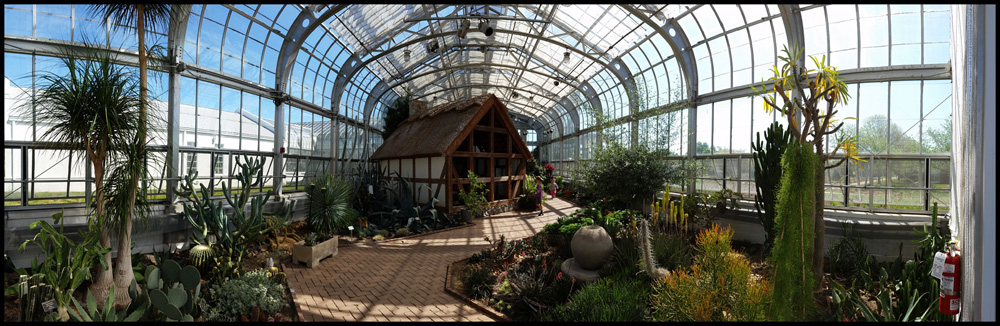This is a detailed panoramic photo of the interior of a large, sophisticated greenhouse with an arched, silver metal frame and walls and roof made entirely of panels of windows. The photograph is bordered by a thin black line and prominently features a small wooden shed with white square siding positioned at the back. The greenhouse floor is laid with red bricks in a sideways pattern, creating a charming walkway through the space. Various desert plants, including cacti, succulents, and a ponytail palm, are planted in beds and planters along the sidewalls. A red fire extinguisher is visible hanging on one wall. Through the greenhouse windows, trees and an adjacent white building can be seen outside, adding to the picturesque view. This decorative and elegant greenhouse appears to be designed for visitors, with its clear glass structure allowing an unobstructed view of both the interior plants and the exterior scenery.